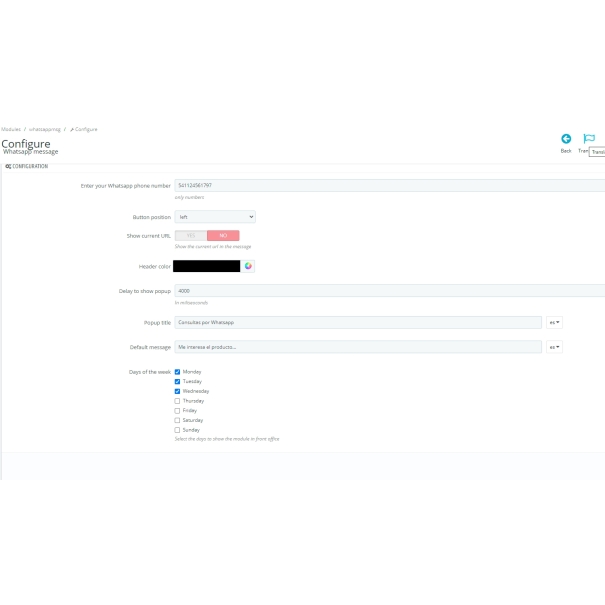The image is a detailed screenshot of a configuration page for a website, possibly for setting up WhatsApp messaging integration. The photo is landscape-oriented and features a white background with internal borders separating various sections.

At the top of the page, there are three small category labels separated by slashes in a grey font, but they are too tiny to be legible. Below these labels, the page title reads "Configure WhatsApp Message". On the right-hand corner, there is a back button icon—a blue circle with a white arrow inside it, accompanied by the text "Back" underneath and a blue flag icon next to it.

Directly beneath the heading, there is a white, long, rectangular section labeled "Configuration" (though the text is small and somewhat hard to read). Within this section, there are several fields and options:

1. A header prompts the user to "Enter your WhatsApp phone number," accompanied by a long, grey input box for the phone number.
2. An additional field, challenging to decipher, includes a drop-down menu for selecting an option.
3. A segment labeled "Show current something," featuring a yes/no toggle switch where the "No" option is highlighted in red.
4. Another box obscured by a grey, redacted mark.
5. Three more input fields for further configuration details.
6. A list of days—Monday, Tuesday, and Wednesday—displayed vertically, each with a checkbox next to it. The checkboxes for these three days are filled out in blue with a white check mark, indicating they are currently selected.

This configuration page offers a variety of settings for customizing WhatsApp messaging functionality on the website.